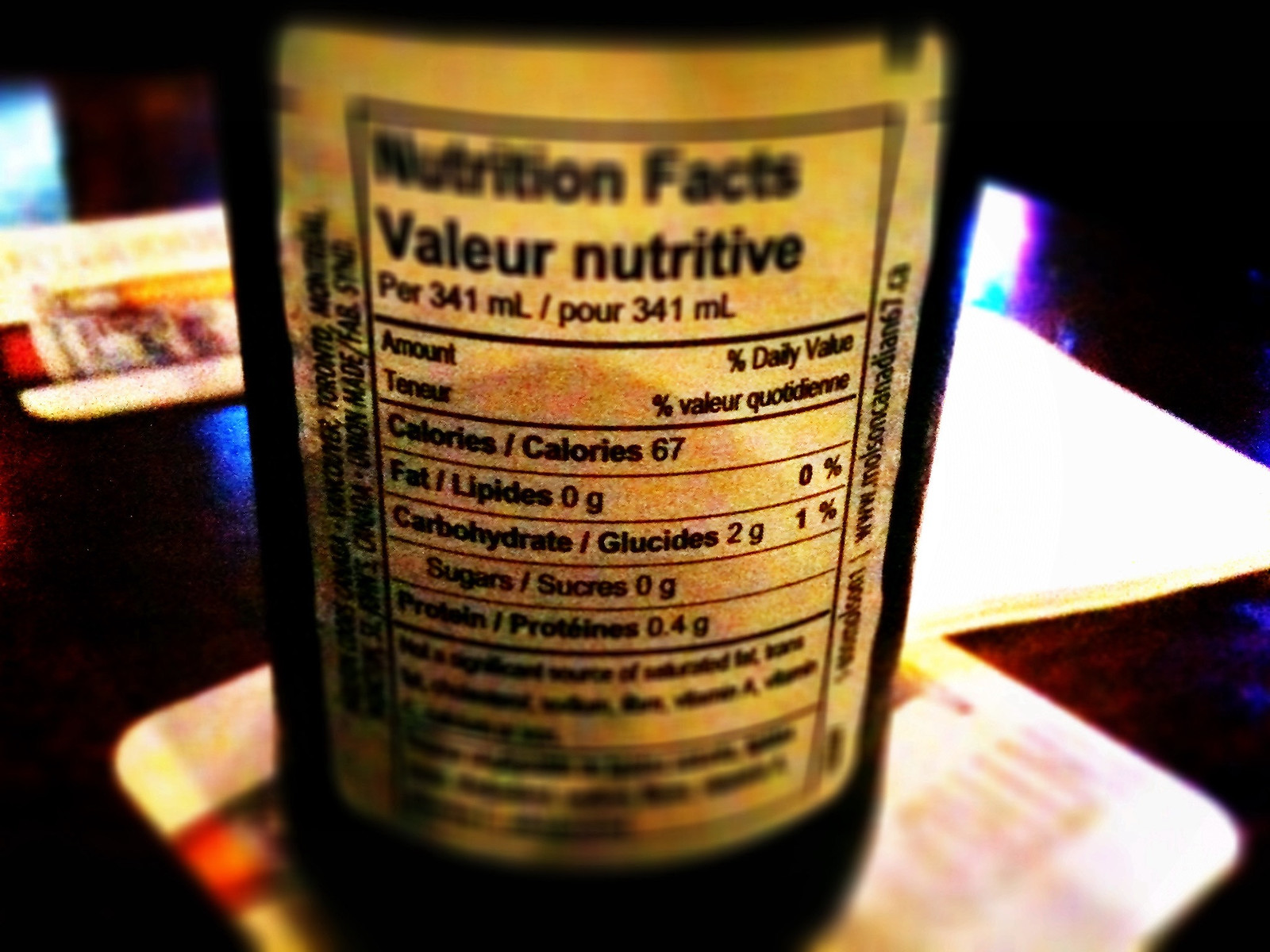This image showcases the back of a consumable product, specifically focusing on the white label that displays nutritional information. The label features a box labeled "Valeur Nutritive," indicating it is likely from a French-speaking country. Within this box, details such as calories, fat, carbohydrates, sugars, and additional nutritional content are listed. The image has a slight blur at the top and bottom, which obscures some of the text, making it challenging to read certain details clearly. Despite the blur, the central portion of the label remains legible, providing insight into the product's nutritional values.